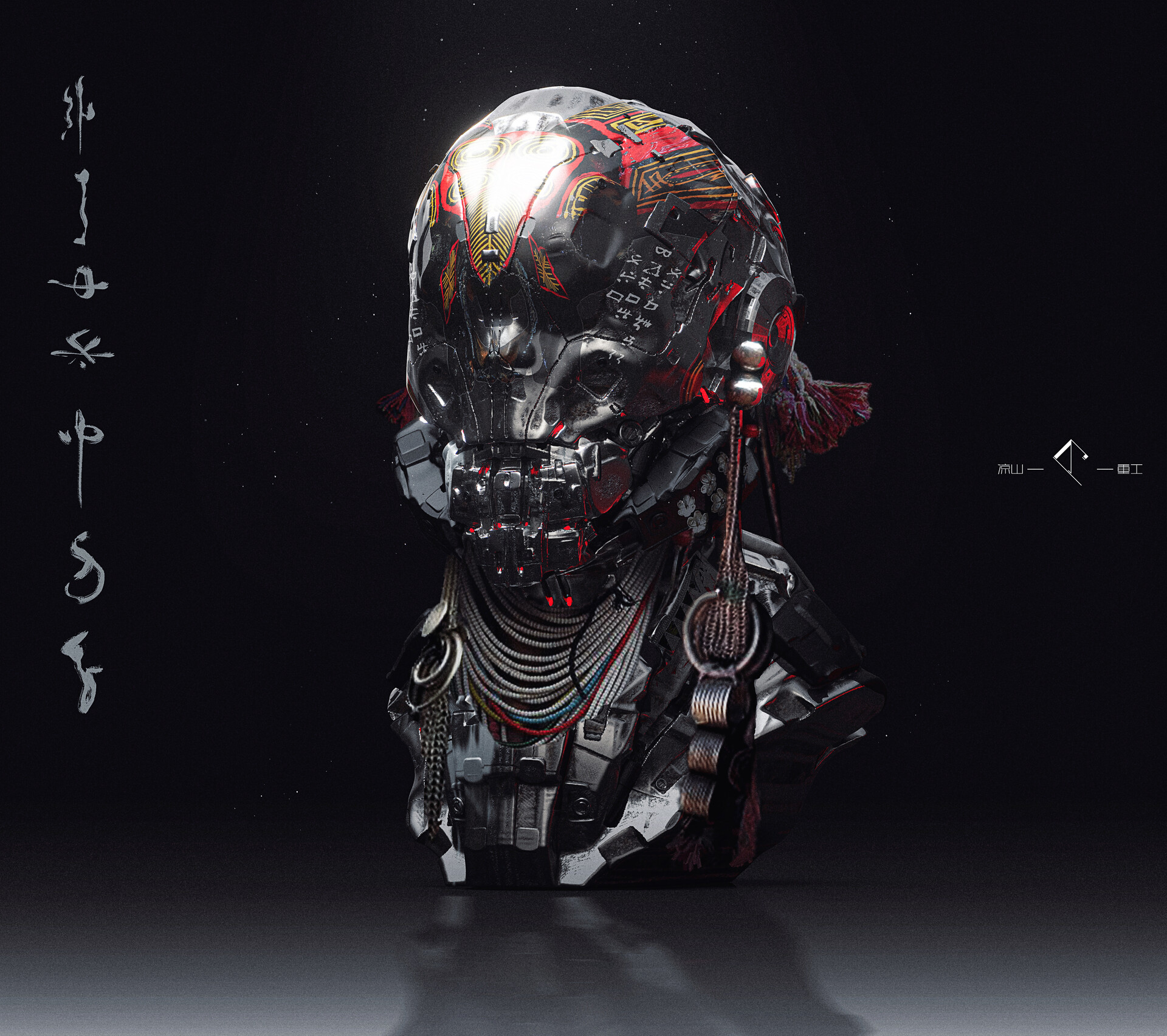In the center of a large, square image with a mostly black background and a gray surface at the base, there is a detailed, photorealistic rendering of a futuristic, robotic head, which appears to also function as a helmet. This imposing headpiece is constructed from black and red metal, with intricate designs in white and gold adorning the forehead, and features a pointed design. The robotic eyes and sharp, mouth-like features contribute to its intense, mechanical appearance. 

Hanging from the head is a tassel-like rope, and around the neck and extending to the upper chest are numerous silver chains, interspersed with colorful beads in blue and red. The head appears mounted on a stand that includes elements resembling arms and a breastplate covering the collarbone and shoulders, emphasizing the upper body structure of the armor. 

On the left side of the image, seven vertical, gray symbols stand out against the black background, while on the right side, a sequence of unfamiliar characters—resembling "A-W", a central design, a dash, and "B-I"—adds a sense of enigmatic foreign script to the scene. The background's void-like quality enhances the stark, highly detailed presentation of this futuristic, mechanical headpiece.